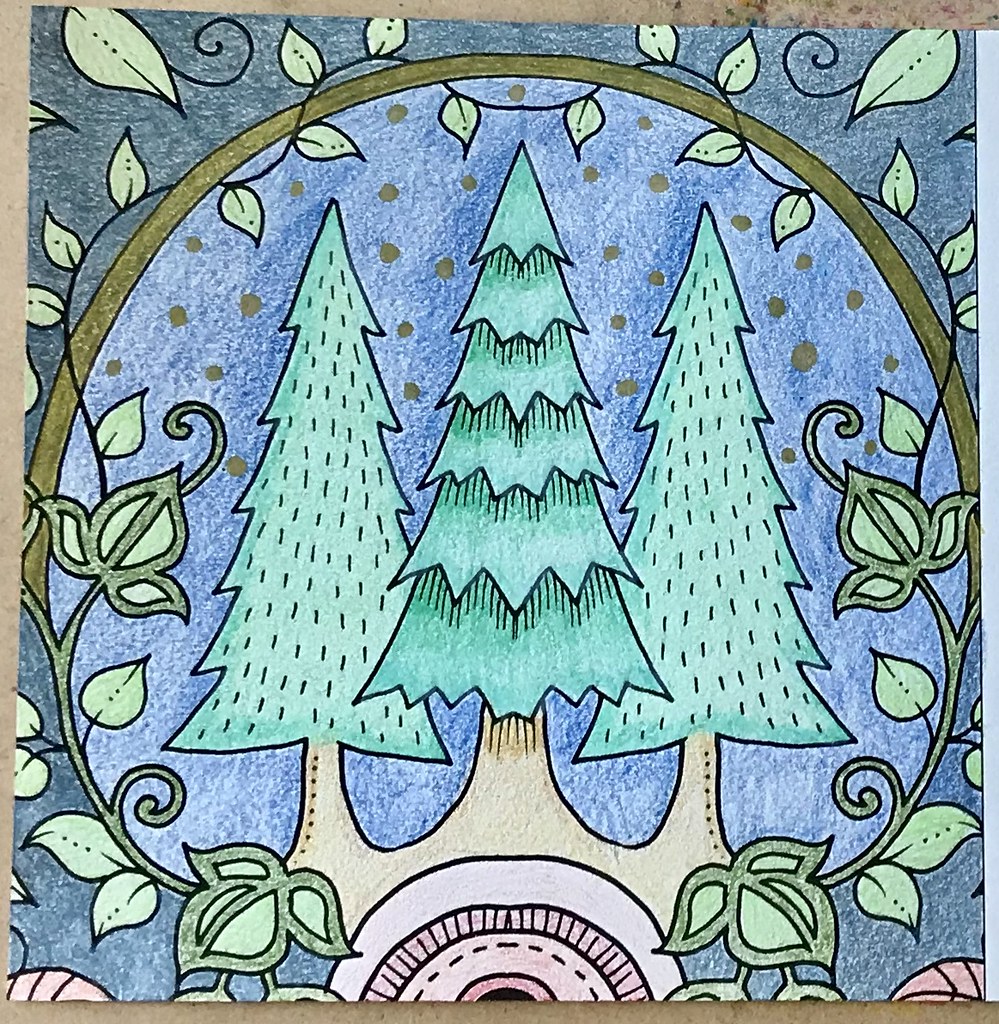A vibrant child's coloring page showcases three evergreen trees prominently in the center, their trunks intricately colored brown and their foliage a lush green. The bases of these trees are interconnected, symbolizing unity. These trees stand on a white circular platform adorned with red accents, giving the image a festive feel. Encircling the trees is a ring-like shape, also green, which seems to be a motif of intertwining vines, adding a sense of natural harmony to the composition. The background is artistically painted in gradients of blue, punctuated by shimmering gold dots scattered around the trees, adding a magical touch to the scene.